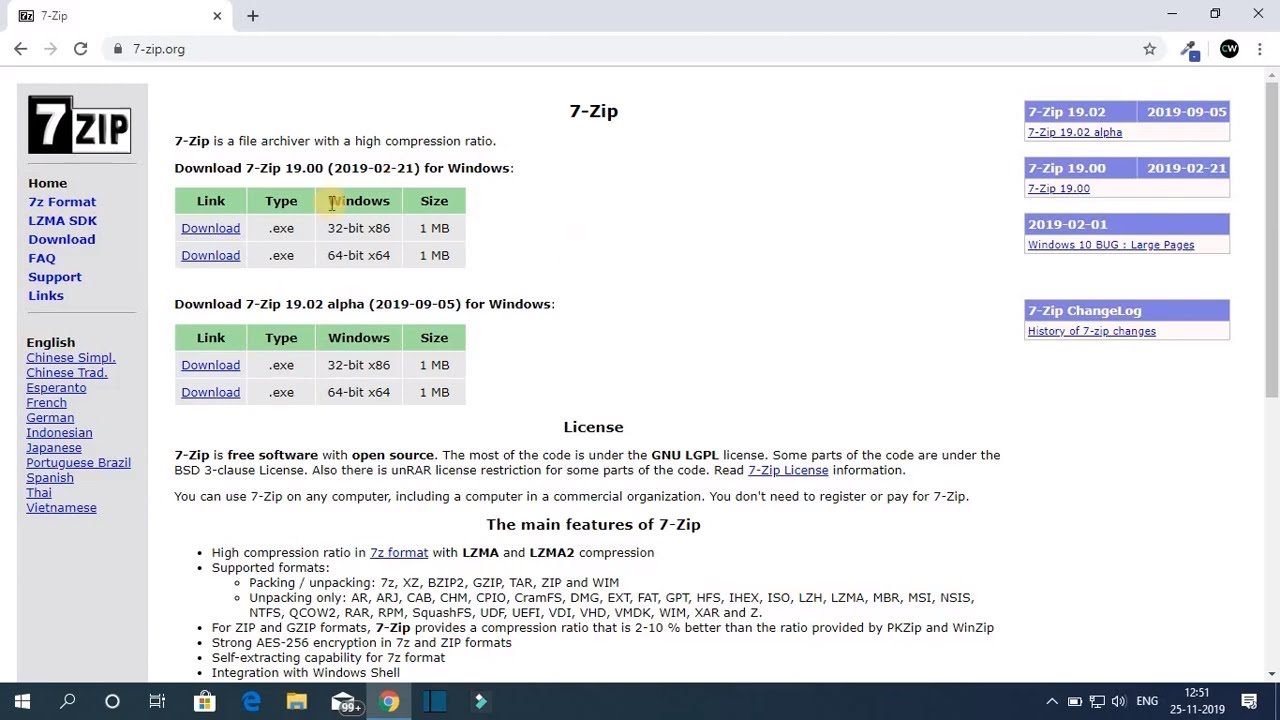The image captures the homepage of 7zip.org displayed on a laptop screen. The website prominently features the 7-Zip logo, which consists of a white number "7" inside a black box followed by "zip" in black text against a white background. Below the logo, the page states that 7-Zip is a file archiver with a high compression ratio. It offers detailed download options for 7-Zip versions 19.00 (dated 2019-02-21) and 19.02 alpha (dated 2019-09-05), both available for Windows. The page also includes the licensing agreement and an overview of 7-Zip's main features. 

To the left of the homepage, a menu bar is visible. To the right, there are hyperlinks for downloading different file versions. The laptop's Windows taskbar is at the bottom of the screen, showcasing icons from left to right: Windows Start menu, search, Cortana, battery/charging indicator, Windows Store, Microsoft Edge, File Explorer, Mail (displaying 99+ unread messages), Google Chrome, Notepad, a right arrow, and finally an up arrow representing additional system tray icons. Further right are indicators showing power connection (indicating the device is a laptop connected to a monitor), sound at 66%, language set to English, the date and time as 12:51 PM on 25-11-2019, and a notifications icon.